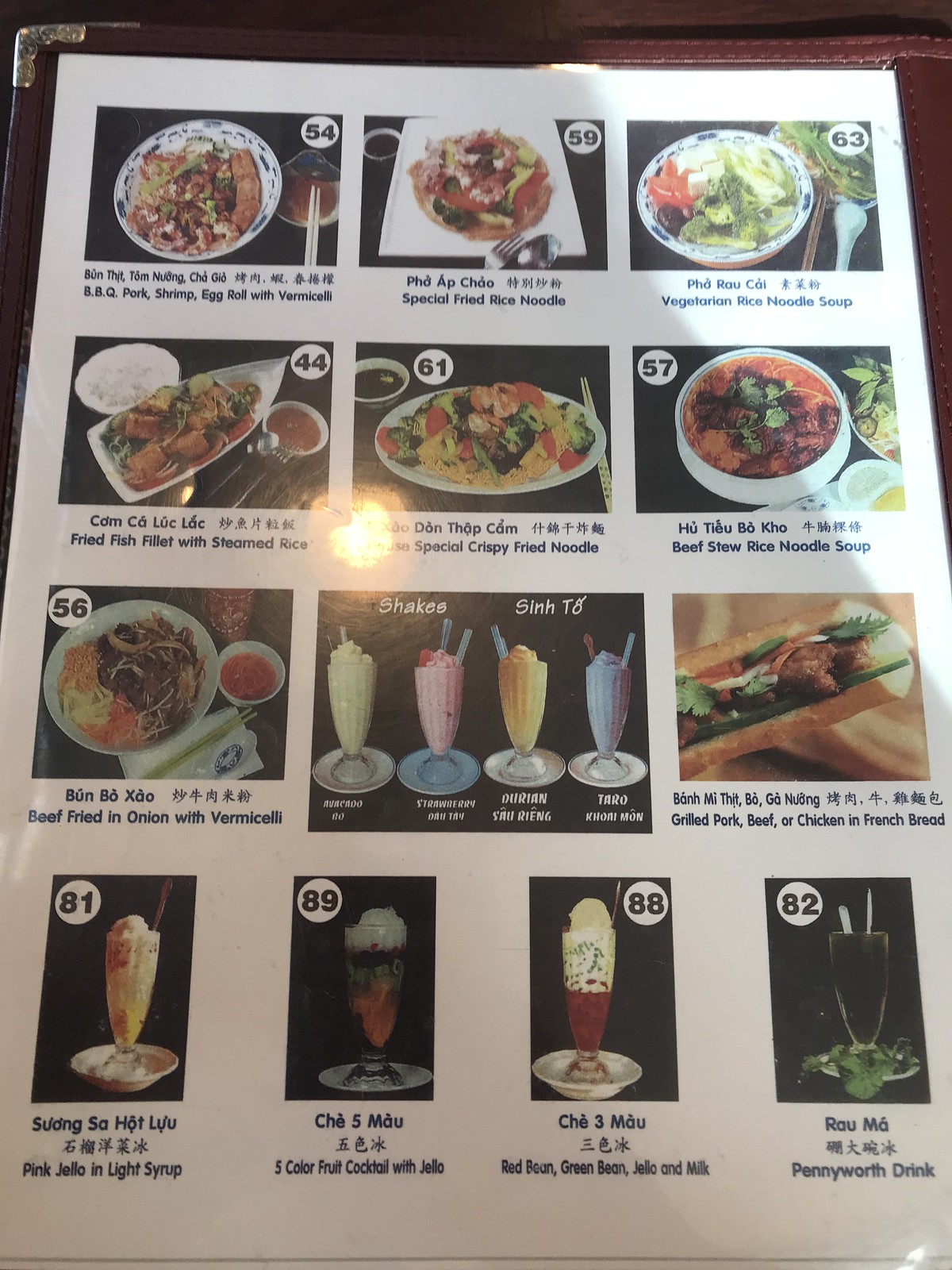This vertical, rectangular image features a menu predominantly encased in a brown border, which extends from the midpoint of the left edge, across the top, and slightly down the right side. The menu rests on a brown table, and in the upper left corner, there's a small silver piece. The menu itself is white and organized into three horizontal rows of images, followed by one row of four vertical images, each depicting different dishes against a black background, except for one.

Each image is marked with a number inside a white circle located in various positions. In the first row, the images are numbered 54, 59, and 63 respectively from left to right. The second row has images numbered 44 on the left, 61 in the center, and 57 and 56 sequentially to the right. Two images in this row lack numbers. The final row has images numbered 81 (left), 89, 88 (right), and 82 (left).

All dishes are served on white plates or in white bowls. The first image of the top row displays a plate with blue decorations and small text indicating it is something like "pork, shrimp, egg roll with something." A drink with a straw is positioned next to it. The second image shows a dish on a white rectangular plate, while the third has something green and red.

In the second row, the first image shows a small white bowl in the top left, the second has a bowl with food pointing to the upper right corner, and the third depicts a bowl containing a liquid. The fourth image showcases a circular plate with chopsticks positioned underneath on the right side, with a visible glare affecting the image.

The one image without a black background features a white bowl containing red food labeled "Beef Stew, Rice Noodle Soup." Below this, another image shows a large bowl and a small bowl of food with chopsticks underneath, labeled "Beef Fried in Onion with Vermicelli." One more image displays four milkshakes in varying colors: vanilla, strawberry, yellow, and blue. Another image features a hero sandwich on a piece of hero bread, labeled "Grilled Pork, Beef, or Chicken in French Bread."

Each menu item is accompanied by descriptions in both English and Asian writing. The final row holds more milkshakes. The first milkshake is described as "Pink Jello in Light Syrup," presented in a tall milkshake container with a saucer. The subsequent milkshakes, though harder to read, appear similar, with the last one containing green leaves and dark liquid. A shadow covers most of the menu, making the upper right corner noticeably brighter.